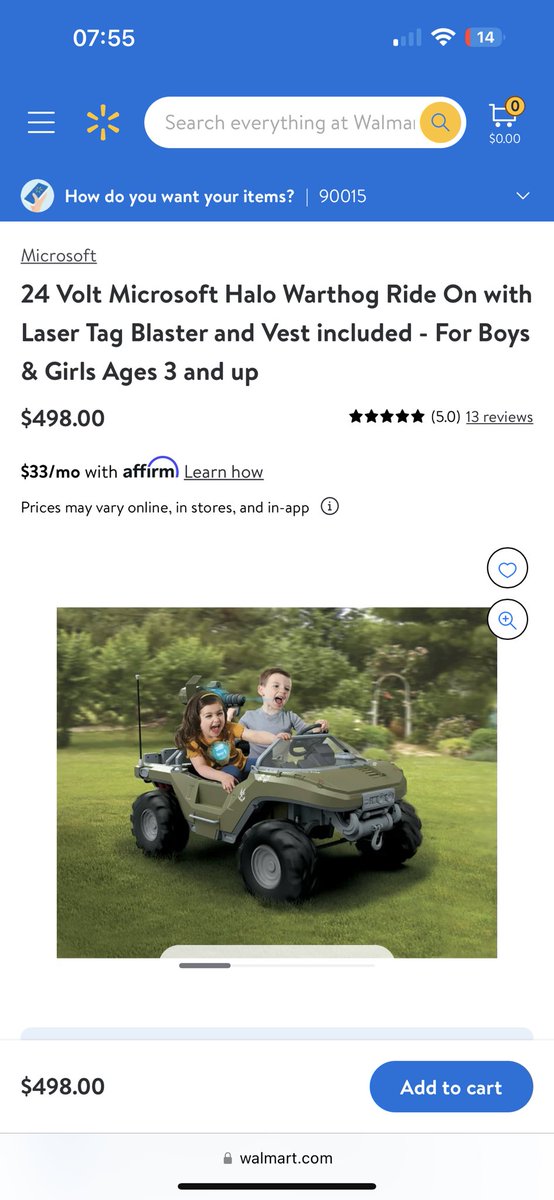This image showcases the Walmart shopping application interface displayed on a cell phone screen. At the very top, a blue banner includes essential system icons: the time on the top left and service and battery indicators on the top right, with the battery indicating a charge of 14%. 

Within this blue banner, from left to right, there are the three horizontal lines indicating a menu drop-down, the Walmart logo icon, a search bar, and a shopping cart icon. Beneath this banner, there is a section displaying the delivery options linked to the postal code "90015," with an expandable arrow for additional options.

Below these navigation elements, the product details for a "24 Volt Halo Warthog Ride-On with Laser Tag Blaster and Vest Included" are prominently shown. This ride-on toy, suitable for boys and girls aged 3 and up, is priced at $498. Additionally, there's a financing option available at $33 per month through Affirm, with a link to learn more about the terms. A disclaimer notes that prices may vary online, in stores, and within the app.

An image of the product follows, displaying the green, battery-operated ride-on cart modeled after a Jeep from the video game Halo. Directly beneath the image, the price of $498 is reiterated. Finally, there is a prominent blue "Add to Cart" button with white text, facilitating easy purchase.

This detailed caption comprehensively describes the elements and layout of the Walmart shopping app's interface as seen in the provided image.